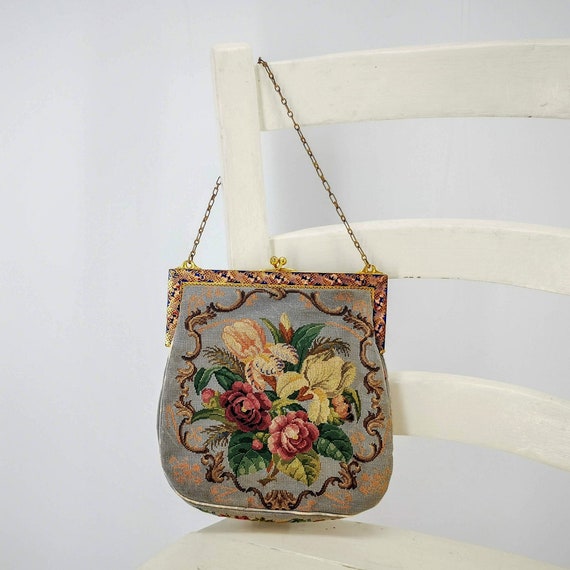The image depicts an old-fashioned purse hanging on an off-white wooden chair with a backrest consisting of three horizontal slats with slightly curved arches. The purse features a golden chain shoulder strap and a shiny gold clasp in the center. The top of the purse is adorned with a jeweled, mauve-colored, sequined pattern. The body of the purse has a faded light blue base framed by an octagonal border with rust or orange accents on the corners. The central design is a bouquet of various flowers, including maroon, red, yellow, and peach blossoms with green leaves, all surrounded by intricate brown swirls and thin branches that add detail to the floral arrangement. The overall appearance of the purse suggests it is quite outdated, contributing to its old-fashioned charm.